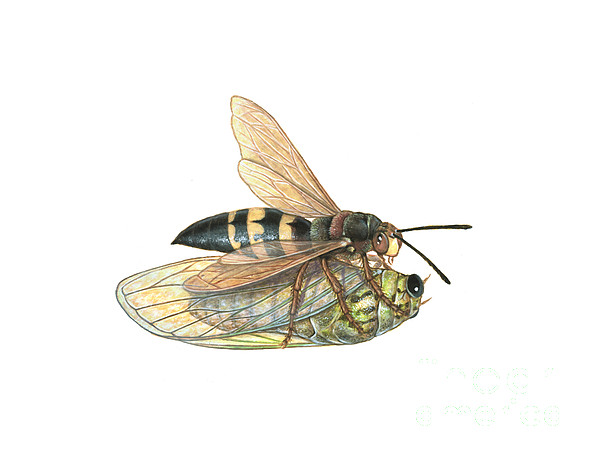This finely detailed illustration from a science textbook captures a dramatic interaction between a cicada and a wasp. The cicada, lying on its back, displays its medium green body with intricate dark green stripes and light green wings. Its head is green with spots of orange and yellow, surrounded by tiers of darker green dots and black spots near its black pupils. Meanwhile, the wasp straddles the cicada, appearing to attack with its three legs wrapped tightly around the cicada's body. The wasp has an eye-catching black abdomen punctuated by alternating orange and black stripes down to its stinger. Its thorax transitions in color from olive to brown to black, culminating in a brown head with orange in the middle and brown compound eyes. The wasp’s golden-tan wings fan outward, and its long black antennae stretch forward, adding to the lifelike intensity of the scene.